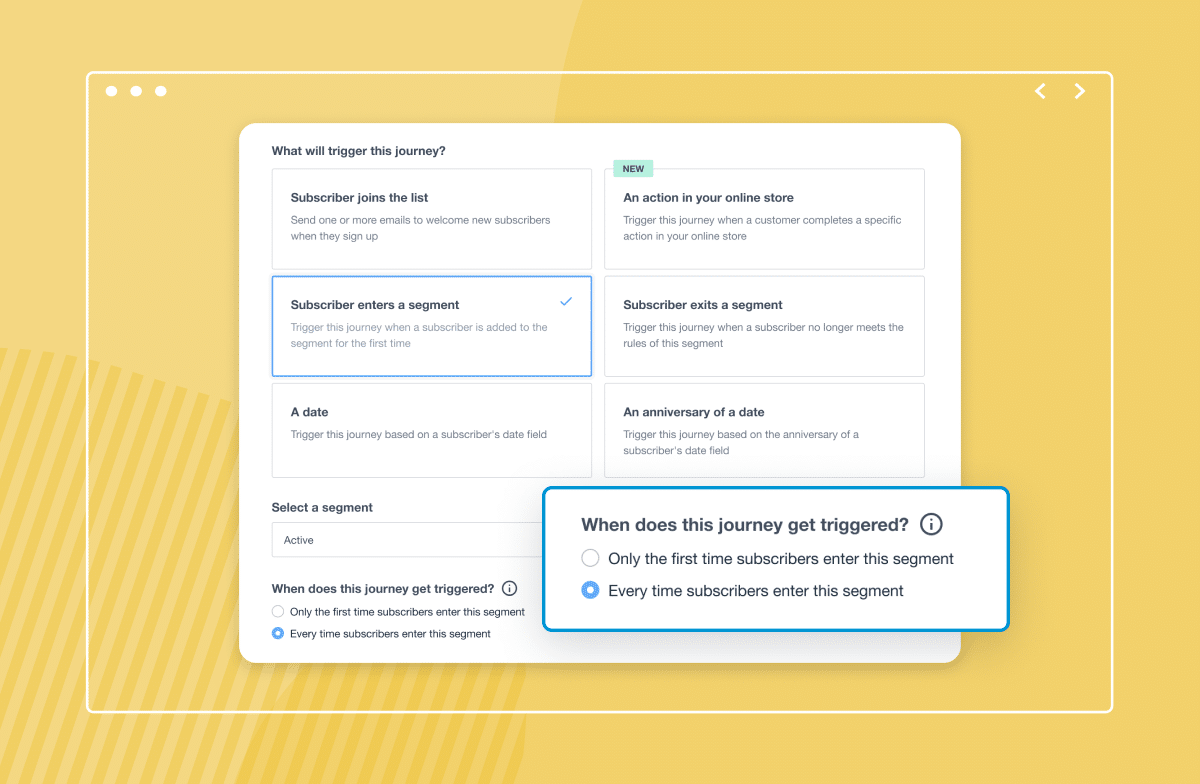Here is a clean and descriptive caption for the image described:

---

The image features a medium yellow background with a central white square containing black text that reads, "What will trigger this journey?" Below this text, there are several options in separate squares, each detailing different triggers:

1. "Subscriber joins the list"
2. "Subscriber enters a segment" - outlined in blue 
3. "A date"
4. "New" - inside a rectangle 
5. "An action in your online store"
6. "Subscriber exits a segment"
7. "Anniversary of a date"

Below these options, there is explanatory text: "Trigger this journey based on the anniversary of a subscriber's date field." In a blue-outlined rectangle, the question "When does this journey get triggered?" is posed. 

This section offers two options:
1. "Only the first time subscribers enter this segment" - indicated by an empty circle 
2. "Every time subscribers enter this segment" - indicated by a filled blue dot

To the left of the options, it is reiterated: "When does this journey get triggered? The answer is every time subscribers enter this segment."

---

This structured caption clearly outlines the visual and textual elements of the image, providing detail and clarity on the content presented.